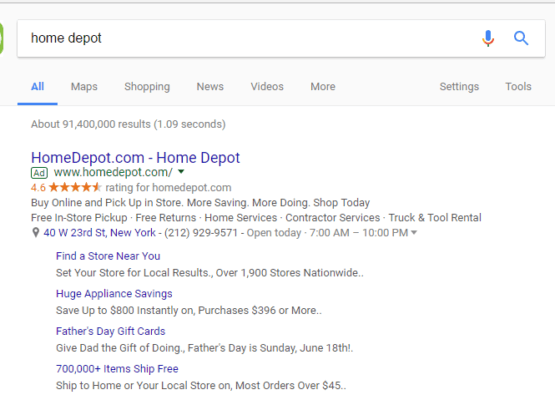The image is a screenshot of a Google search result for "Home Depot." At the top, there is a standard Google search interface, with a microphone icon to the left and a magnifying glass icon to the right. The navigation bar below includes tabs labeled 'All' (highlighted and selected), 'Maps,' 'Shopping,' 'News,' 'Videos,' and 'More,' along with 'Settings' and 'Tools' on the far right.

The search results indicate "About 91,400,000 results (0.09 seconds)" just below the navigation bar. The first result is a clickable link in blue text to Home Depot's official website, followed by a clickable URL: www.homedepot.com. The entry displays a 4.6-star rating for Home Depot's site and promotes various services such as "Buy online and pick up in store," "More saving, more doing," "Shop today," "Free in-store pickup," "Free returns," "Home services," and "Contractor services."

Additional information includes the store's address on "40 W 23rd Street, New York," followed by a blue phone number "212-929-9571," and the hours of operation, "open today 7 a.m. to 10 p.m." Furthermore, there are links for finding a nearby store, huge appliance savings, Father's Day gift cards, and a note on "700,000+ items free," indicating local results spanning over 9,000 stores nationwide. An advertisement promotes savings of up to $800 on purchases of $396 or more, encouraging shoppers to give "the gift of doing," with a reminder that Father's Day is Sunday, June 18. There is also a note about free shipping on most orders over $45.